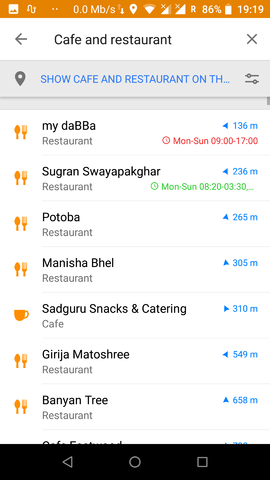This image is a screenshot of a device displaying search results for cafes and restaurants. The top bar of the screen shows the time as 9:19 AM, with an 86% battery charge, strong Wi-Fi, and cellular signal indicators, along with a location services icon. The background of the web page is white, and the header reads "Cafe and Restaurant," accompanied by a location icon. Below, blue text instructs "Show cafe and restaurant on," followed by several icons. The search results list includes the following establishments: IDABBA, Sun Grand, Protoba, Manisha Bell, a cafe offering snacks and catering, and two additional restaurants. Each restaurant is marked with a spoon and fork icon, while the cafe features a coffee cup icon.